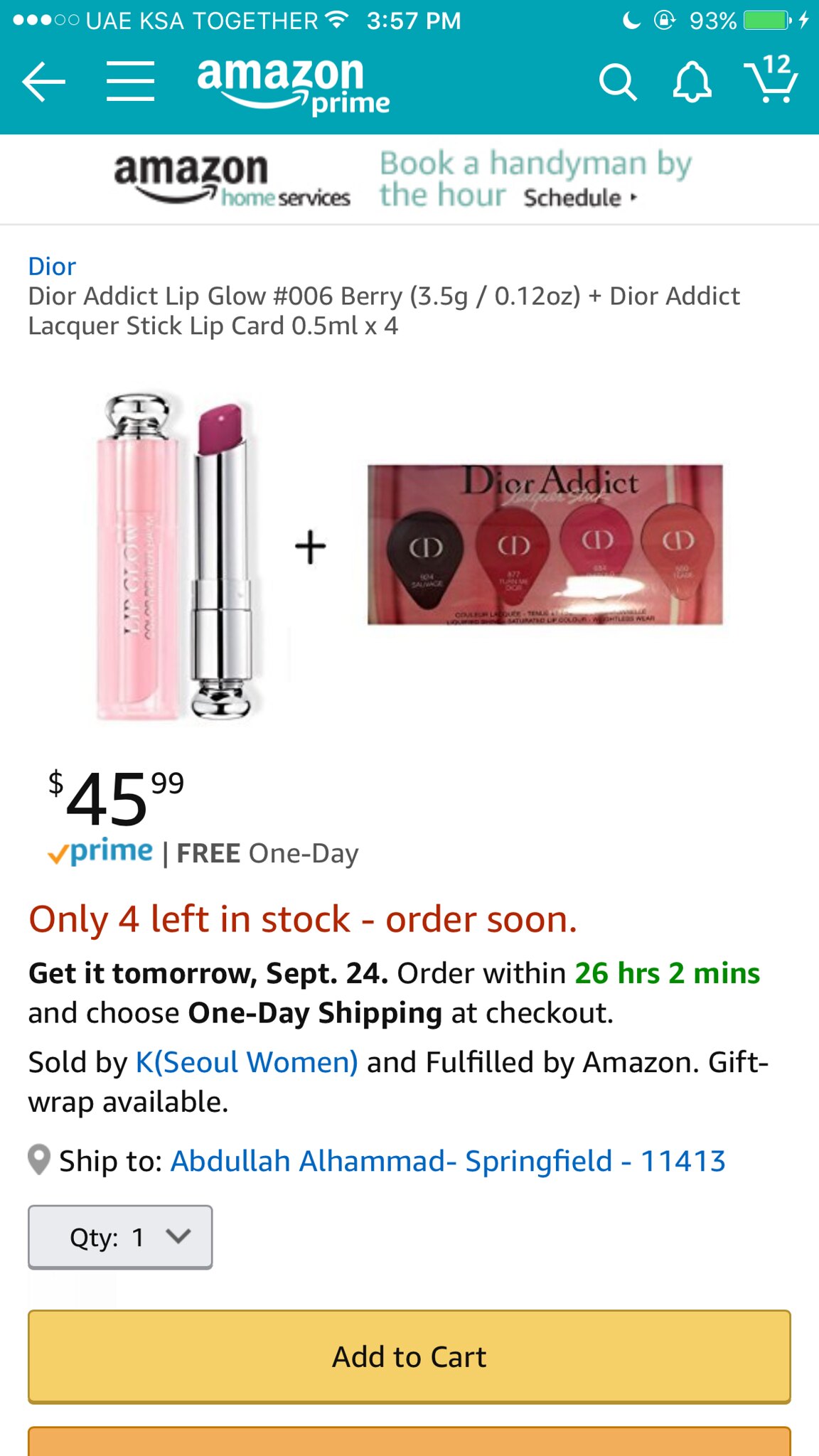The image is a screenshot of an Amazon product page taken from a mobile phone, evident by the presence of typical smartphone icons at the top. Dominated by a teal-colored header with white symbols and the Amazon logo, the listing appears to be from the UAE. The product showcased is the Dior Addict Lip Glow Berry, priced at $45.99, with only four left in stock. The lipstick tube features a reflective silver shaft and the lip glow itself is a deep pink, or magenta color. To the left of the lipstick, there is what seems to be a pink skinny tube of perfume with a small glass cap. The product page includes options to select the quantity and add it to the cart, highlighted by a large yellow "Add to Cart" button at the bottom. The image also features colors such as blue, white, black, red, silver, yellow, and cream. Additionally, text such as "home services" and "book a handyman by the hour" are visible in the header.